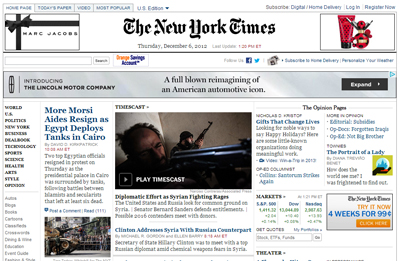The image depicts the homepage of The New York Times website. At the top of the page, navigation options are visible, including links labeled "Today's Paper," "Video," "Most Popular," and "U.S. Edition." There is also a drop-down arrow allowing users to switch from the U.S. Edition to other regional editions. The prominent New York Times logo, written in cursive, is displayed below the navigation bar, alongside the date "Thursday, December 6, 2012."

An advertisement for Marc Jacobs features a white box adorned with a black gift bow. Below this ad, viewers can find a search bar and options to follow The New York Times on Facebook and Twitter. Further down, there is a promotional section for "Introducing the Lincoln Motor Company, a full-blown reimagining of an American automotive icon."

Headline links such as "More Morrissey Aids Resign as Egypt Deploys Tanks in Cairo" and "Gift that Changes Lives" are displayed in blue text, indicating they are clickable. The main cover image showcases a man holding a gun and another man appearing to be in pain. Additional images include one of a bulldozer on a street.

Various sections are listed, including "World," "U.S.," "Politics," "New York," "Business," "Dealbook," and "Technology." The overall design features mostly black text with blue hyperlinks on a white background, creating a clean and readable layout.